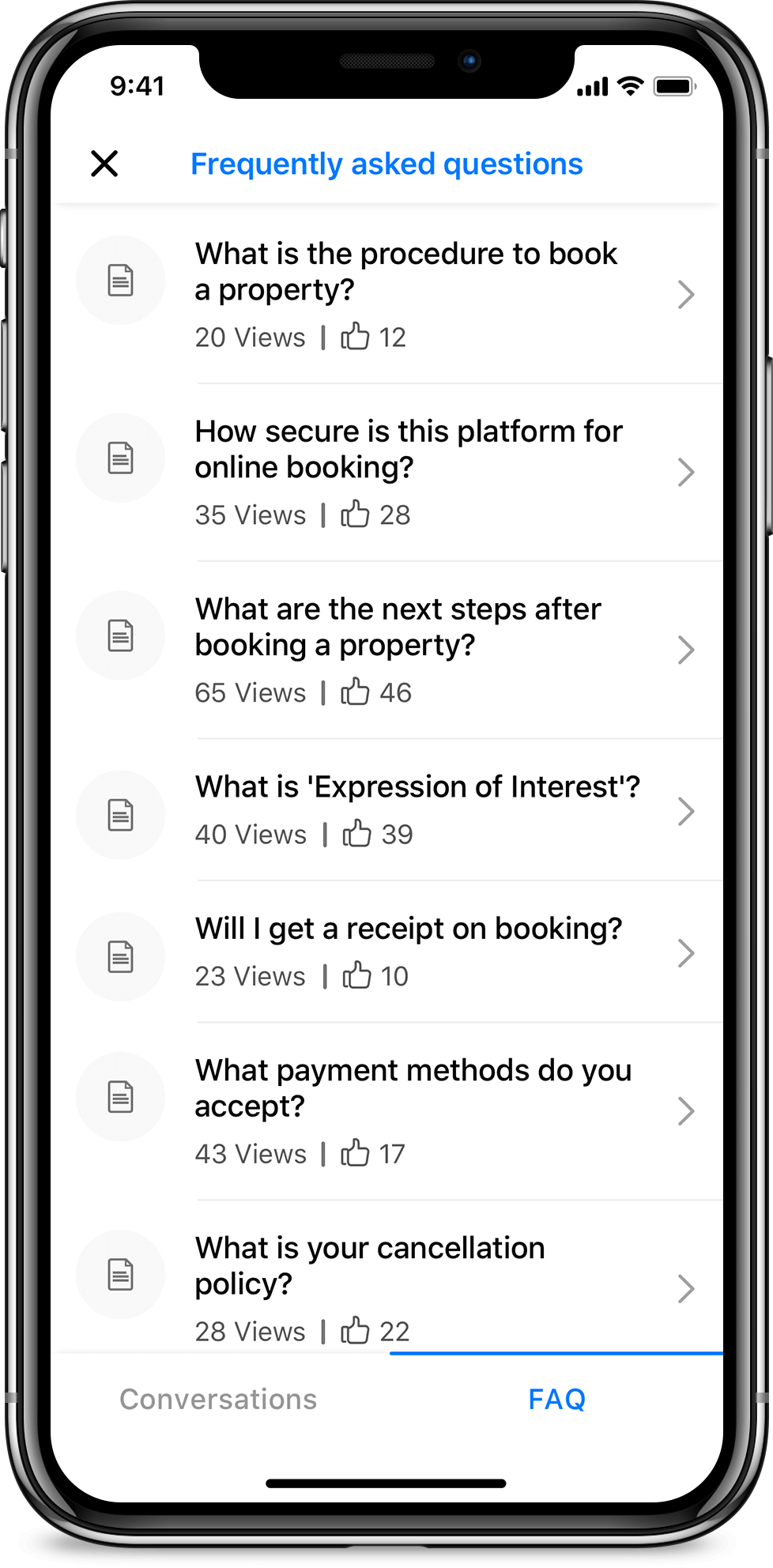The image is a screenshot of a mobile phone displaying a Frequently Asked Questions (FAQ) section. In the top left corner of the screen, the time is shown as 9:41. Adjacent to the time, various status icons can be seen, including signal bars indicating cellular reception, a Wi-Fi symbol, and a fully charged battery icon on the right.

At the center of the screen, in blue text, is the title "Frequently Asked Questions" with a black 'X' to its left, presumably to close the FAQ section. Below this title, there is a list of seven questions, each numbered consecutively from one to seven:

1. What is the procedure to book a property?
2. How secure is this platform for online booking?
3. What are the next steps after booking a property?
4. What is expression of interest?
5. Will I get a receipt booking?
6. What payment methods do you accept?
7. What is your cancellation policy?

Each question is accompanied by details showing the number of views and the number of likes it has received, indicating the popularity and frequency of inquiry for each question.